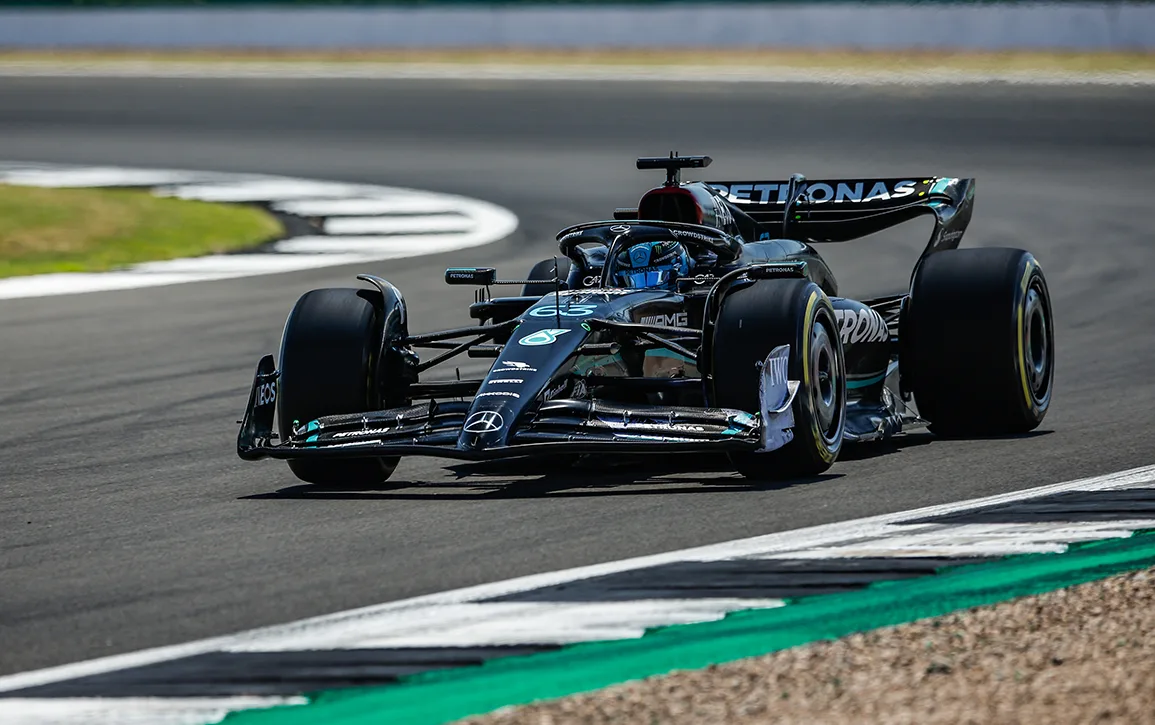The photograph captures a sleek, black Mercedes Formula One race car emblazoned with various white decals, including the prominently displayed word "PETRONAS" on the tail fin and the number 63 on the front of the car, just ahead of the driver. The car is expertly maneuvering around a right-hand turn on a race track, bordered by distinct white and black lines marking the track's boundaries. The driver's helmet, adorned in black with mirrored, reflective goggles, is partially visible above the cockpit. Patches of grass to the left and gravel to the bottom right frame the racing scene, emphasizing the car's swift movement on the curving track.